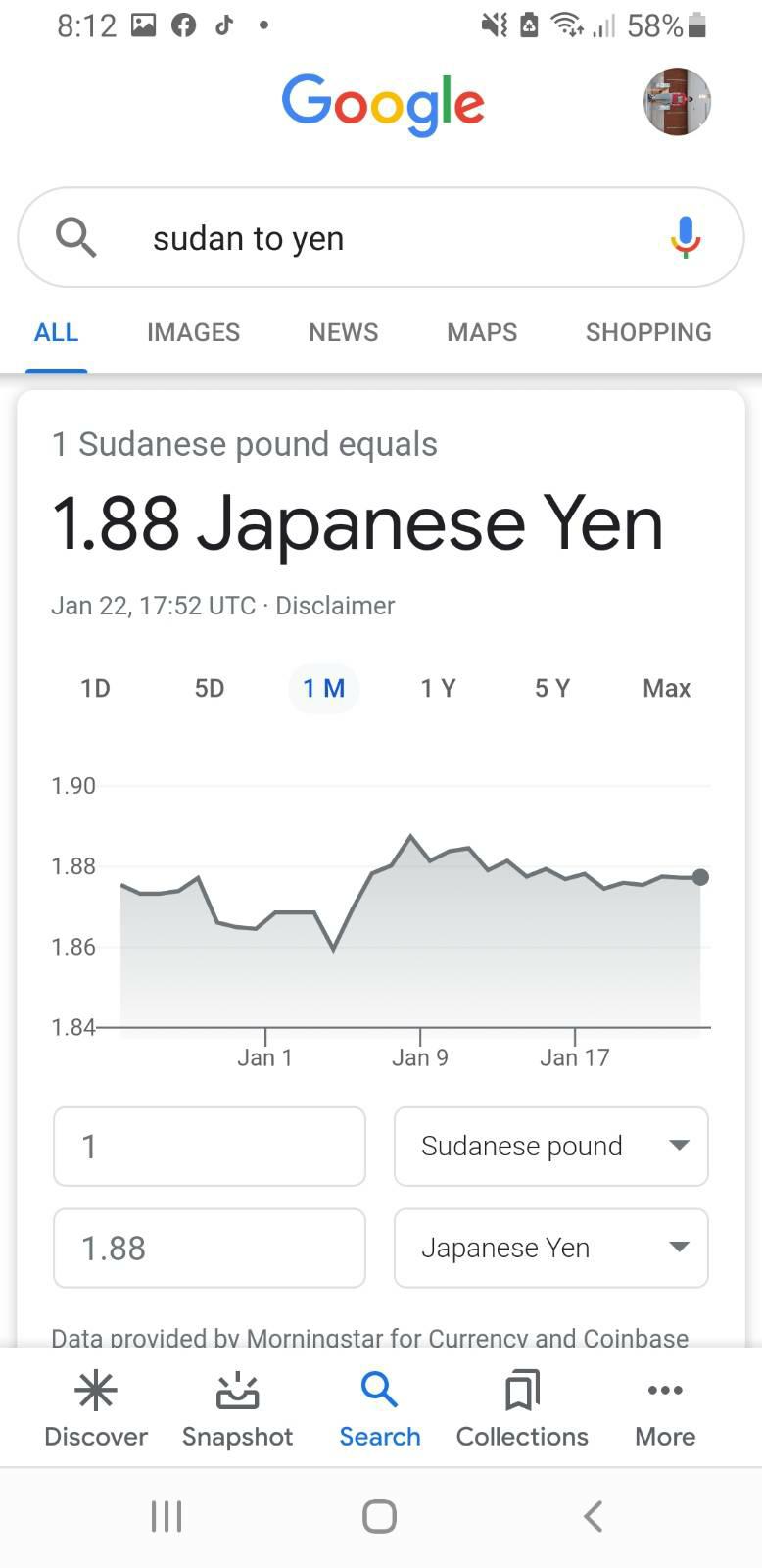Detailed Descriptive Caption:

The image displays a white background featuring a smartphone screen with the time displayed as 08:12 and a battery level of 58%. The top of the screen prominently shows the Google search bar, which includes a magnifying glass icon on the left and a microphone icon on the right. Just below, there's a user's profile picture. In the search bar, the entered query reads "Sudanese pound to yen."

Below the search bar, there is a horizontal navigation menu containing options like "All," "Images," "News," "Maps," and "Shopping," all highlighted in blue. The main content area of the screen shows the current exchange rate, stating "1 Sudanese pound equals 1.88 Japanese yen" with the timestamp of January 22nd, 17:52 UTC, along with a disclaimer about the data.

There is a graph depicting the exchange rate trend over time, with selectable time frames marked as 1D, 5D, 1M (highlighted in blue), 1Y, 5Y, and Max. The line graph below covers specific dates such as January 1st, January 9th, and January 17th, with the corresponding exchange values marked as 1.87, 1.89, and 1.88 yen respectively. The vertical axis on the left of the graph shows exchange rate levels at intervals of 1.84, 1.86, 1.88, and 1.90 yen.

Additional interface elements include rectangular buttons labeled "1 yen" and "Sudanese pound," along with another rectangular display showing "1.88" and "Japanese yen." At the very bottom, the data source is attributed to Morningstar for currency data and Coinbase.